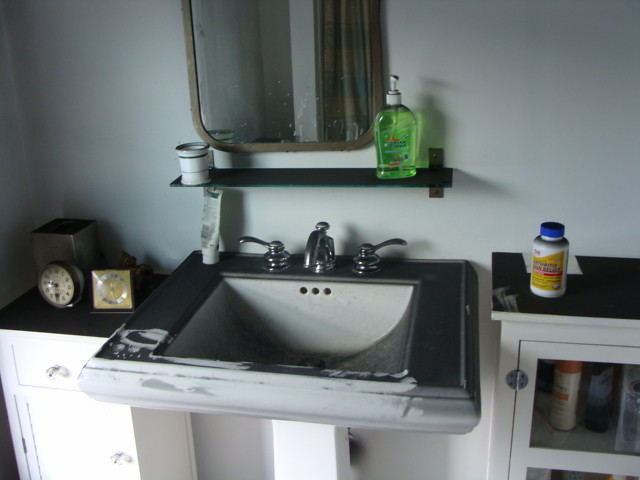This photograph captures a vintage bathroom featuring a prominent self-standing pedestal sink. The sink, which appears to be made of white cast iron or ceramic, has its top surface painted black. Over time, the black paint has worn away in areas on the front and left side, revealing the original white surface beneath. The pedestal itself is approximately six inches wide and has a rectangular or square shape, extending down to the floor.

To the right of the sink, there is a white cabinet with glass doors, inside of which several bottles and jars are visible. One of these appears to be a white bottle with a blue top and a yellow label, possibly containing vitamins. On the left side of the sink is another white cabinet featuring round, crystal-like knobs. Atop this cabinet are one or two clocks, adding to the eclectic and nostalgic charm of the bathroom's decor.